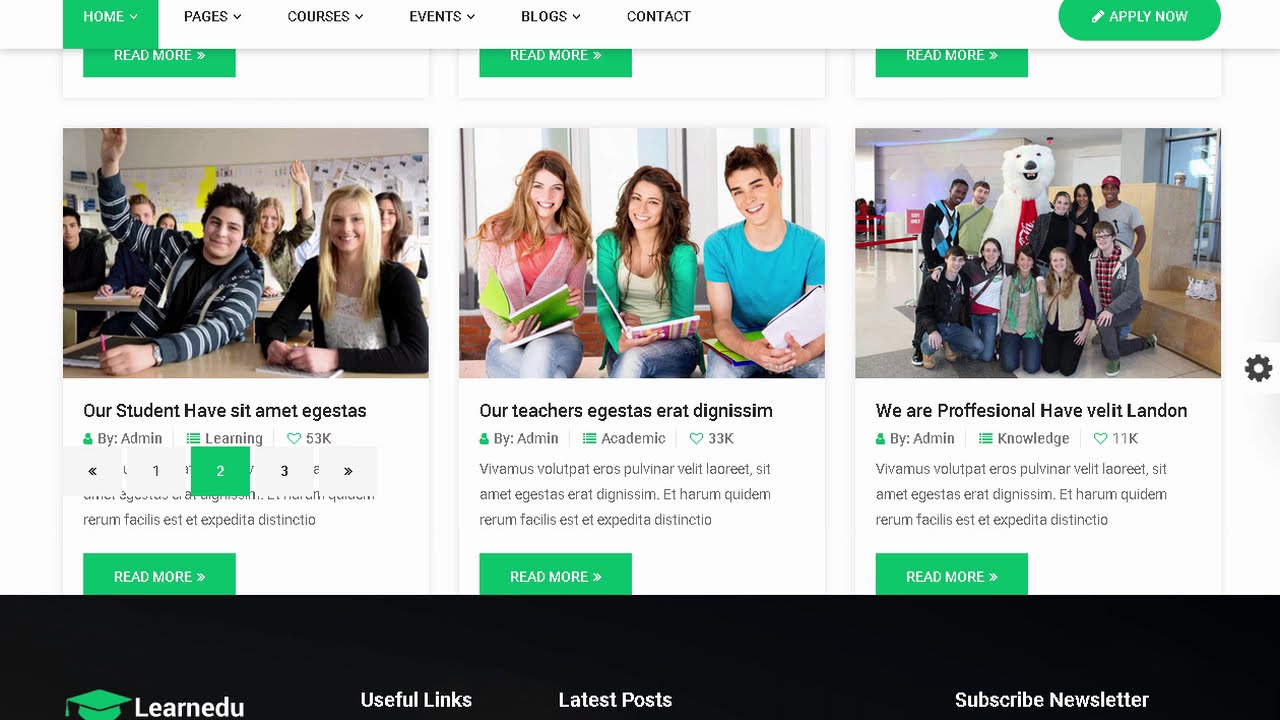This is a screenshot of a classroom website featuring a gray header at the top with six tabs labeled: Home (outlined in green), Pages, Courses, Events, Blogs, and Contact. Each tab has a small arrow indicating a dropdown menu, and in the upper right-hand corner, a green 'Apply Now' button with white text stands out. Below the header, the page is divided into three sections, each showcasing a different photograph. The leftmost image depicts a classroom scene with students eagerly raising their hands, captioned "Our Students Have Met eGestures" with a rating system below. The center image features two women and a man holding a book, accompanied by the caption "Our Teachers eGestures, You Read." The rightmost image shows a group of people posing with a polar bear, highlighting a communal atmosphere. The background is primarily white, maintaining a clean and professional look. At the bottom of the page, a black footer with white text contains a green graduation cap icon next to the words "LearnEDU" and additional sections labeled Useful Links, Latest Posts, and Subscribe Newsletter.